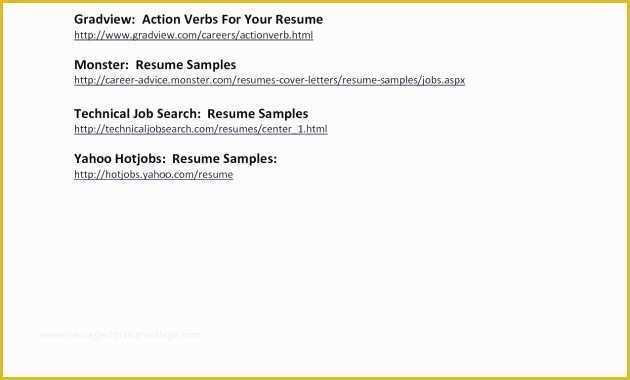The image features a horizontal layout, approximately 50% wider than it is tall, encased in a golden-brown border that surrounds the entire perimeter. The central background within this border is a pristine white, creating a clean and clear canvas for the text.

Starting from the top, there's a bold, black header in a larger font size that reads: "Grand View: Action Verbs for Your Resume," with each word capitalized. This text is notably indented about 10% from the left edge of the image, establishing a consistent margin throughout.

Beneath the main header, the first line of smaller black text contains a website, maintaining the same indentation. After a single line break, the second section begins, featuring another prominent, bold, black text line that reads: "Monster Resume Samples." Following this, there is a corresponding link in a smaller font, continuing the pattern of indentation.

The content continues similarly:
- A space follows the second section.
- The third entry, "Technical Job Search Resume Samples," is again in bold, black, large font with an aligned link in smaller text immediately beneath it.
- Another space precedes the fourth and final section.
- "Yahoo Hot Jobs Resume Samples" is presented in the same bold and large black font, followed by its associated link in smaller text.

Throughout the image, the consistent use of indentation, spacing, and font hierarchies organizes the information clearly, making it easy to follow and visually appealing.